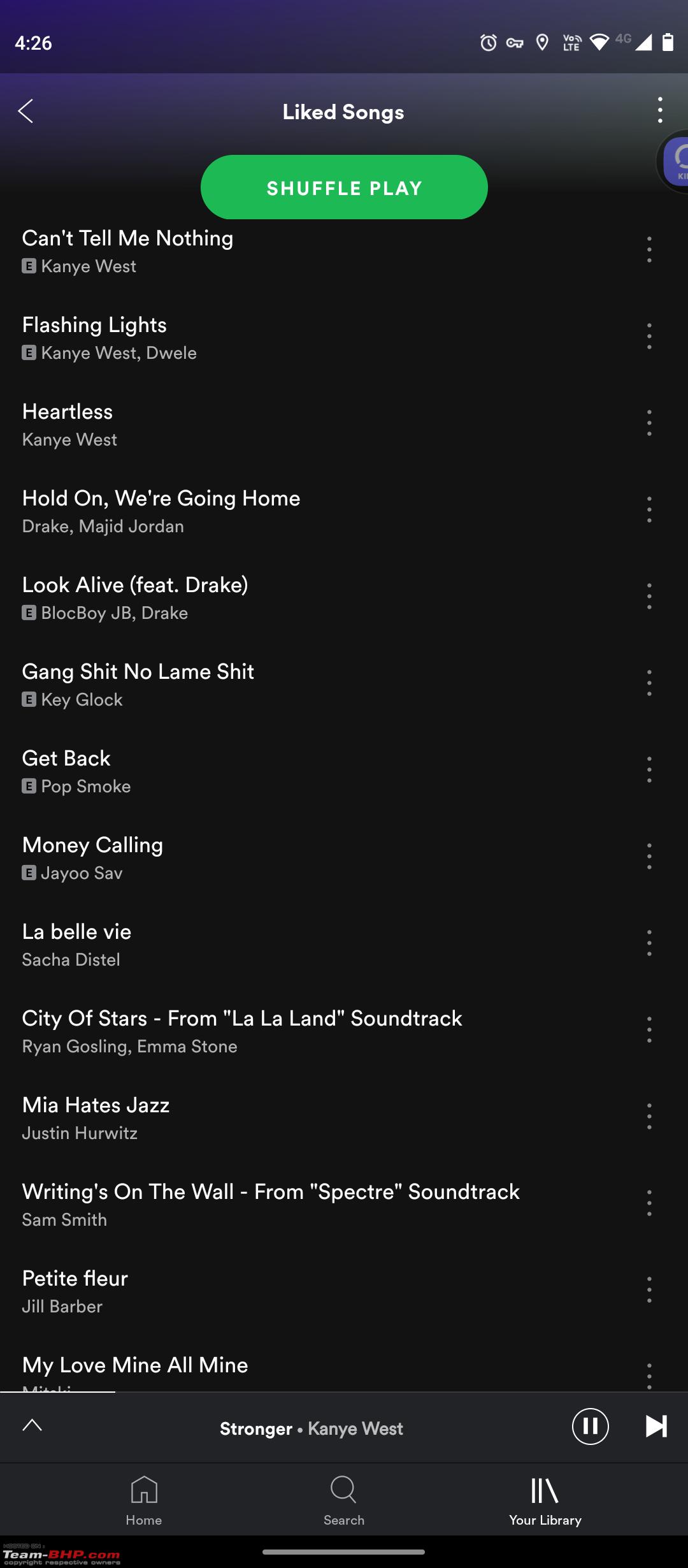This vertical, portrait-mode image appears to be a screenshot from a mobile device, primarily showcasing a list of songs within a music streaming app. The dimensions of the image suggest it is roughly three times as tall as it is wide, making it narrower than most standard smartphone screens. The predominant background color of the image is a very dark black, with headers and footers featuring variations of dark blue and purple hues.

At the very top, the header section is a deep bluish-purple color with white text. On the upper left, the time is displayed as 4:26. To the right, a series of seven or eight icons include an alarm clock as the first, a location pin as the third, a partially filled Wi-Fi icon as the fifth, and finally, a vertical battery icon showing around 80-85% charge.

Below the header, a slightly lighter purple-blue bar displays the title “Liked Songs” in white, centered at the top. On the far left of this bar, a left-facing arrow is present, and on the far right, there are three vertical white dots indicating additional options. Directly underneath this, a green rectangular button with rounded edges states “SHUFFLE PLAY” in white, all-caps text.

The main content displays a list of 14 songs, each formatted with the song title in bold white followed by the artist(s) in a lighter white underneath. Many songs are marked with a white square containing a dark 'E' to denote explicit content. On the right of every song entry, three vertical white dots indicate further actions. The first song listed is "Can't Tell Me Nothing" by Kanye West, followed by other tracks featuring artists like Dwele, Drake, and Key Glock. The artist names are detailed thoroughly, including features and collaborators. The last visible song is "My Love, Mine, All Mine," although the artist's name is cut off, suggesting the list is scrollable.

A footer section at the bottom features a slightly lighter charcoal gray background, showing the currently playing song, “Stronger” by Kanye West, in bold white text centered near the top of this section. To the left, there’s an upward-facing arrowhead, while to the right, icons for pause, and skip forward are displayed. The very bottom row includes navigation options: a house icon labeled "Home" on the left, a magnifying glass labeled "Search" in the middle, and an icon representing books labeled "Your Library" on the right.

Overall, this detailed screenshot provides a comprehensive view of a user's playlist within a music streaming application, complete with navigation, playback controls, and an indicator of the currently playing track.